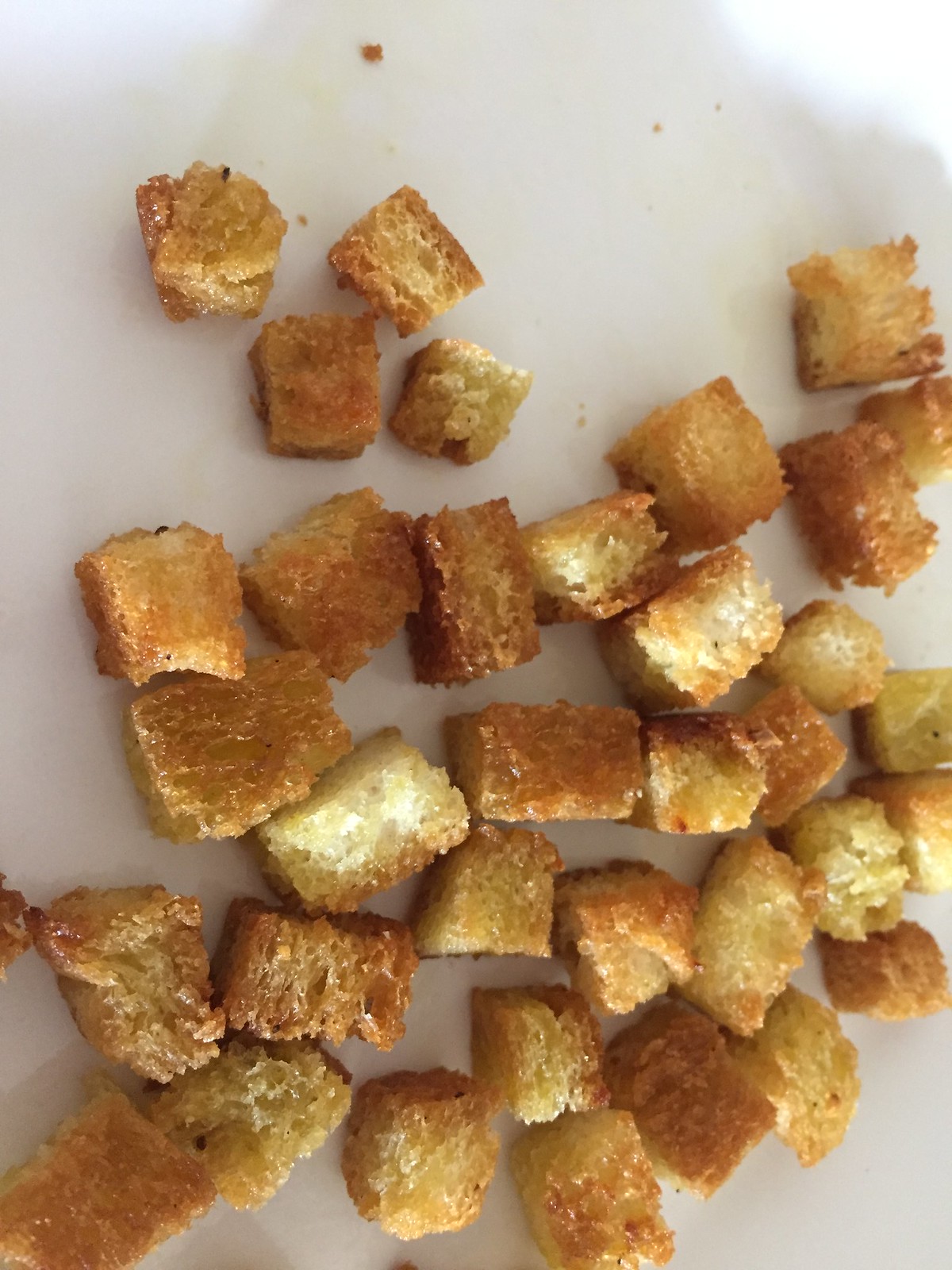This is a color photograph taken in portrait mode, depicting a haphazard pile of golden brown croutons on a white background, viewed from directly above. The croutons are small cubes and rectangles of toasted bread, appearing both light and dark brown. Their texture is crispy and airy, evidenced by visible cavernous regions within the bread. Scattered crumbs and shadows, created by the direct lighting, add to the overall texture and detail of the scene.